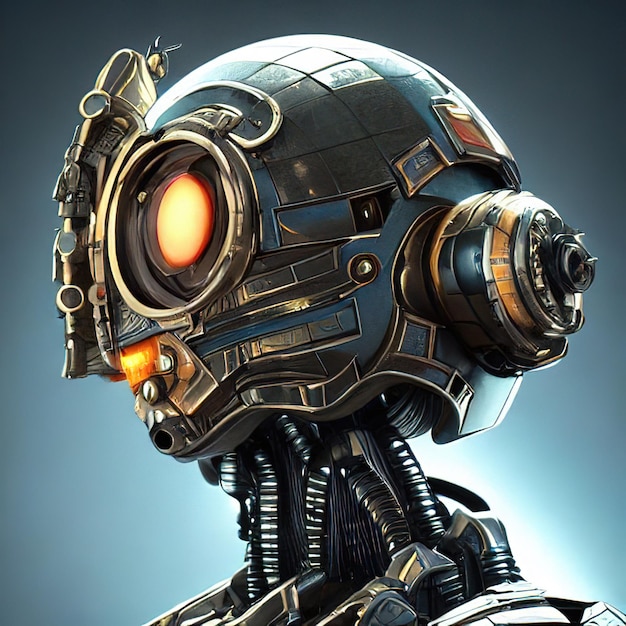This detailed digital art piece depicts the head and neck of a humanoid robot against a blue background that transitions to white. The robot, primarily bluish-silver with accents of dark grey, black, and gold, has a complex assembly made of numerous small pieces. Dominating its face is a single, orange, camera-like eye, encased in a metal ring with a shutter style design and a red center. A solar panel-like structure adorns the top of its helmet-like head. Extending from the left side of its head is a protruding, microphone-like round component resembling an ear, while another tall, silver piece sticks up beside the head on the right. The neck, appearing flexible, connects to the body via numerous cords and cables. An orange or yellow light is set where its mouth would be, enhancing its futuristic look.